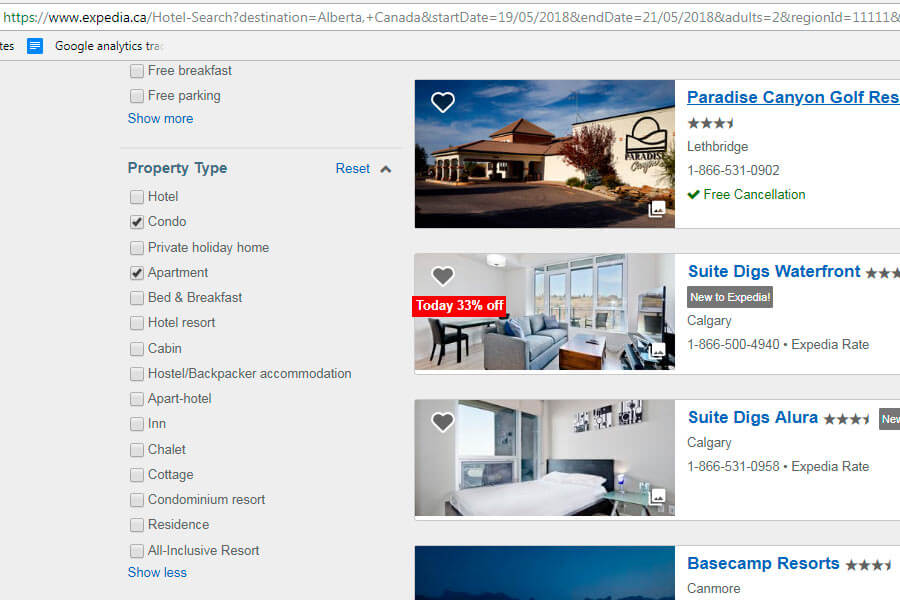This image, sourced from www.expedia.ca, showcases a segment of a web page likely related to property listings. The focal point is a blue box with white lines across it that contains several key pieces of information. Within this box, "Google Analytics" is mentioned, though the context isn't fully clear. Prominent features highlighted include "Free Breakfast" and "Free Parking" with a "Show More" option in red text. 

The category "Property Type" is also featured, with "Condo" and "Apartment" checked off, while other options such as "Hotel," "Bed and Breakfast," "Inn," "Chalet," and "Cottage" remain available but unchecked.

To the right of the blue box, there are four vertically arranged images. Each image includes:

1. **Paradise Canyon Golf Resort**: This entry features a golf resort, though no specific details are given in the image.
2. **Sweet Digs Waterfront**: This listing highlights a waterfront property with a special discount of 33% off for the day.
3. **Sweet Digs Allura**: This entry includes a bedroom picture, indicating that people have favorited it, along with the second listing.
4. **Baseball Resorts in Canmore**: Only a portion of this image is visible, showcasing a sky view, suggesting the website’s layout may require scrolling to view in full.

The overall presentation is indicative of a property listing page, providing various filters and featured properties that users can explore further. Some visual elements, like a scroll button, may be missing or cut off in the captured image.